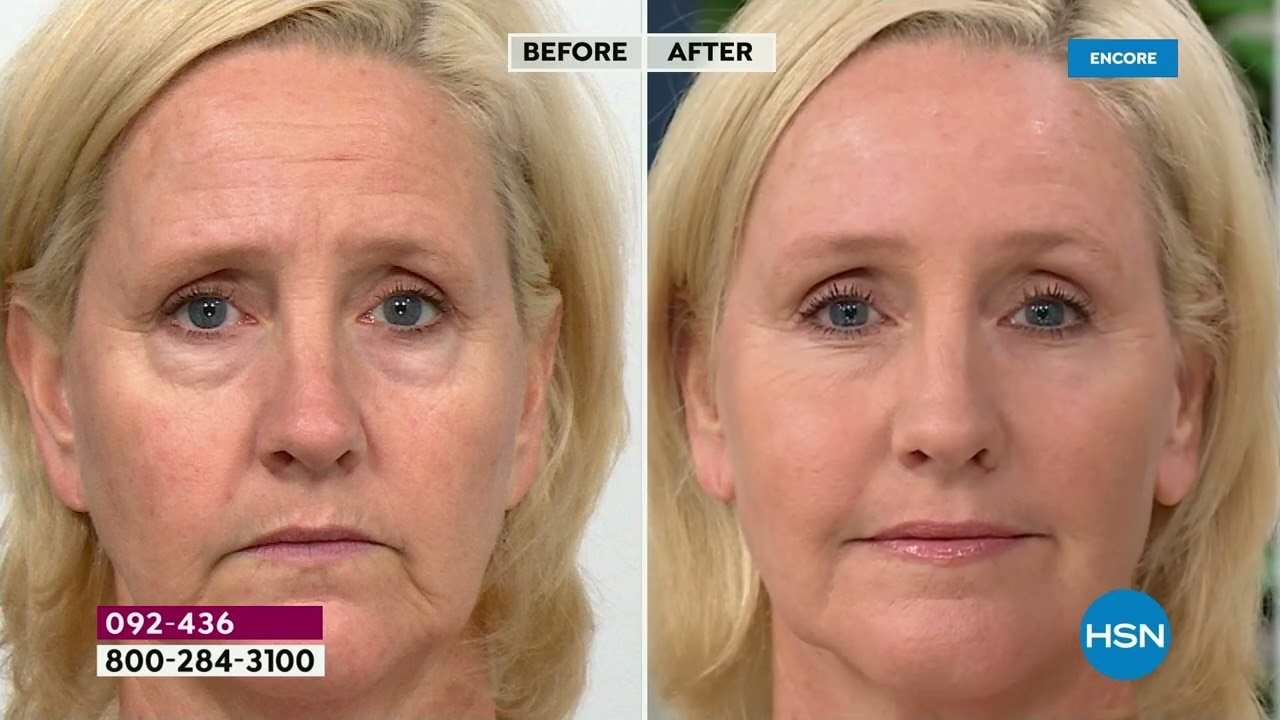This image is a detailed before-and-after photograph of a woman, showcasing the effects of a cosmetic product. The composition features two side-by-side photos: the "before" picture on the left and the "after" picture on the right. In the "before" image, the woman appears to be in her 50s, with noticeable wrinkles on her forehead, crow's feet around her eyes, and dark circles under her eyes. She also has lines around her mouth and prominent bags under her eyes. Her complexion appears uneven, and she is not wearing makeup. In the "after" image, her complexion looks much improved. The wrinkles on her forehead are no longer visible, the crow's feet are barely noticeable, and the dark circles under her eyes have disappeared. Her lips also appear smoother with fewer lines, and she is wearing makeup that enhances her overall appearance.

The text in the image includes a number “092-436-800-284-3100” at the top, with "Encore" at the top right corner, and "HSN" (Home Shopping Network) at the bottom right corner, along with a recognizable logo. The predominant colors in the image are beige, blonde, blue, burgundy, white, black, and green. Both photos indicate that the woman is staring directly into the camera, emphasizing the transformation. The setting and layout suggest this is an advertisement for a beauty or cosmetic product, highlighting the significant visual improvements achieved by the product showcased.